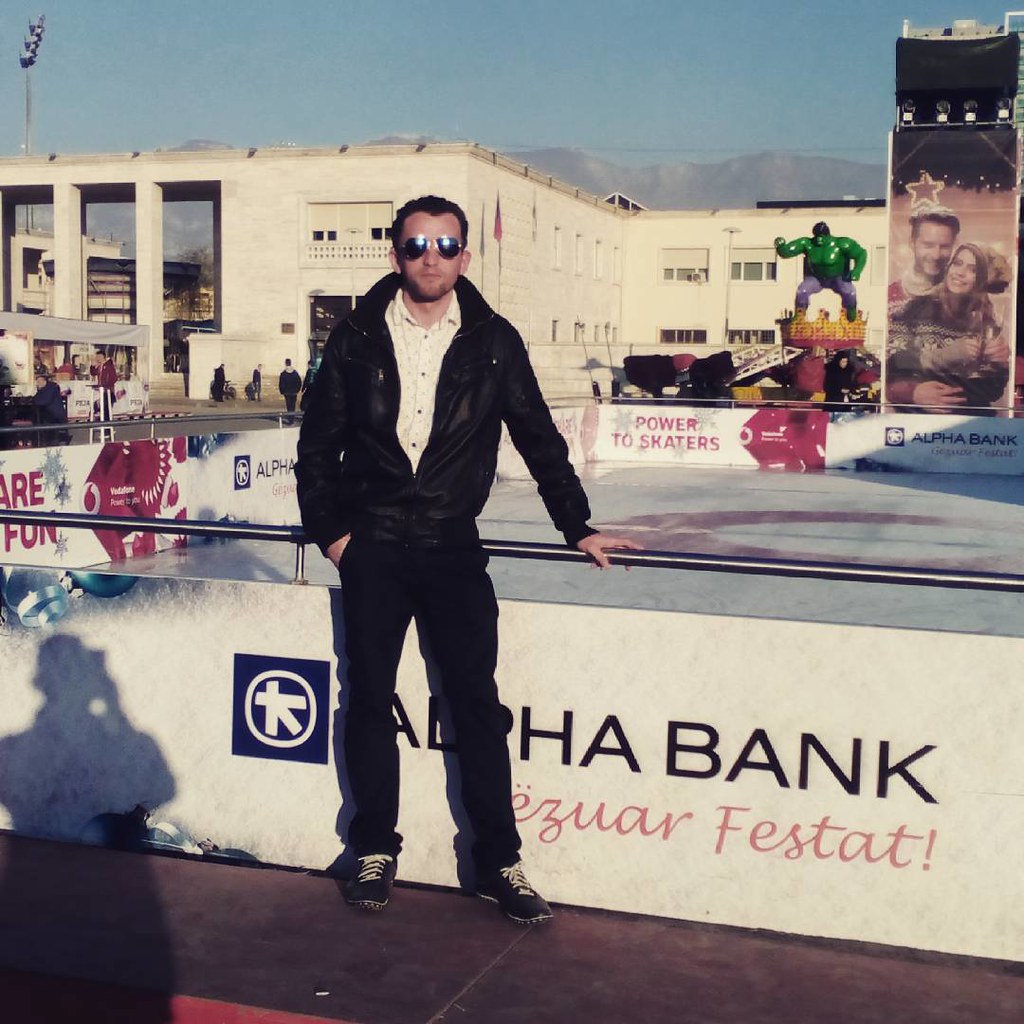A man stands confidently in front of an outdoor ice rink, marked by a low barrier wall with the words "Alpha Bank" and "Power to Skaters" printed on it. He is dressed in a stylish ensemble consisting of a black bomber jacket, a white button-up shirt, black pants, and black shoes with white shoelaces. His look is completed with aviator sunglasses, short brown curly hair, and a goatee. The man's right hand rests on the rail, while his left hand is casually tucked into his pocket. The background reveals a bustling scene with a mixture of people walking, white low buildings, and a striking green statue of the Incredible Hulk, seemingly part of a fairground ride. A mountain range adds a picturesque dimension to the backdrop. Additionally, there's a large photo of a couple and the shadow of the photographer is faintly visible in the bottom left corner.